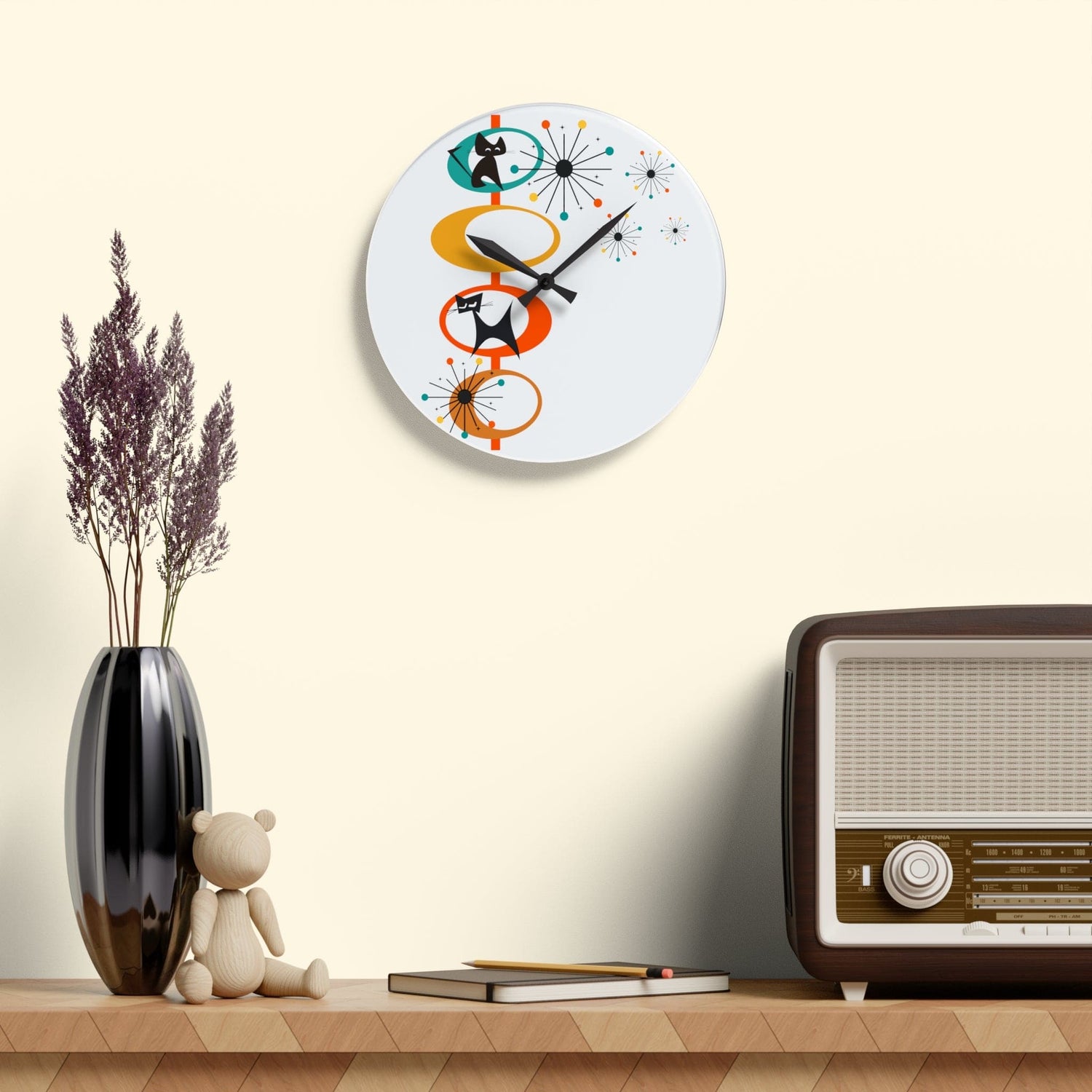The image depicts a detailed 3D render of an indoor setting, showcasing a meticulously arranged scene atop a wooden table or shelf. The wood surface has a patterned design featuring interlocking parallelogram shapes in varying shades. On the left, there is a shiny, dark pewter metallic vase filled with fluffy, pink wildflowers. Nestled beside the vase is a small, articulated wooden teddy bear, sitting and leaning against it. Central to the composition is a brown-covered notebook with a yellow pencil resting atop it. To the right stands an old-fashioned radio reminiscent of a 1940s ham radio, adding a vintage touch.

Above this setup, a unique, white, circular wall clock is mounted on a cream-colored wall. The clock lacks traditional numbers and instead features a series of colorful rings - yellow, red, and orange. Two black cartoon-style cats are situated within the green and red rings respectively. Additional starburst-like designs or atomic patterns embellish the clock, contributing to the whimsical and eclectic aesthetic of the scene. The overall palette and elements suggest a blend of vintage and playful modern design, creating a visually rich and engaging atmosphere.